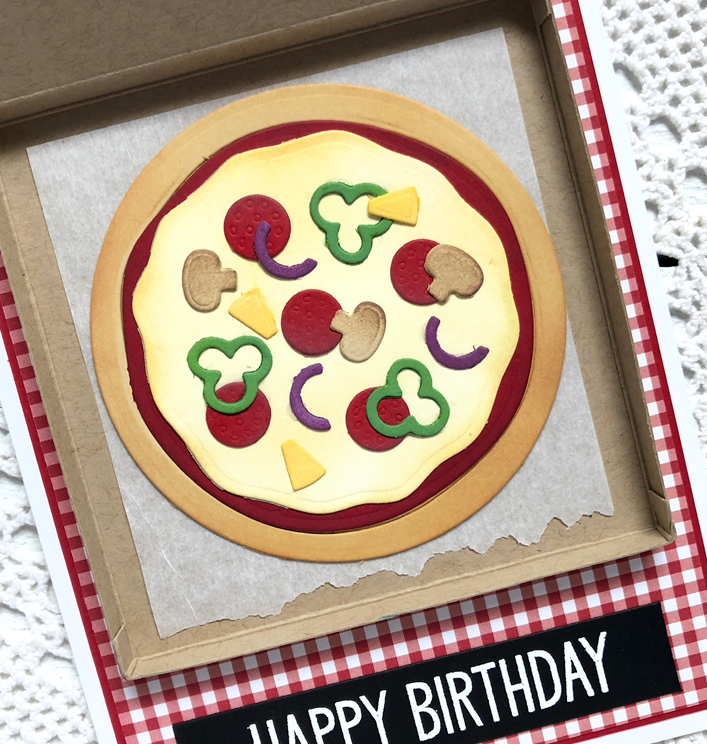The image is of a birthday card featuring a detailed, whimsical depiction of a pizza set in a cardboard box. The centerpiece of the card is a cartoonish, circular pizza made out of paper, complete with playful representations of toppings like pepperoni, onions, green peppers, mushrooms, and pineapple. The pizza rests on a waxy paper inside its cardboard container. This setup sits atop a red and white plaid background, adding a classic picnic vibe. Surrounding this scene is a subtle lace border, giving the card an elegant touch. At the bottom, the message "Happy Birthday" is prominently displayed in white text. This charming card would be an excellent choice for any pizza enthusiast.